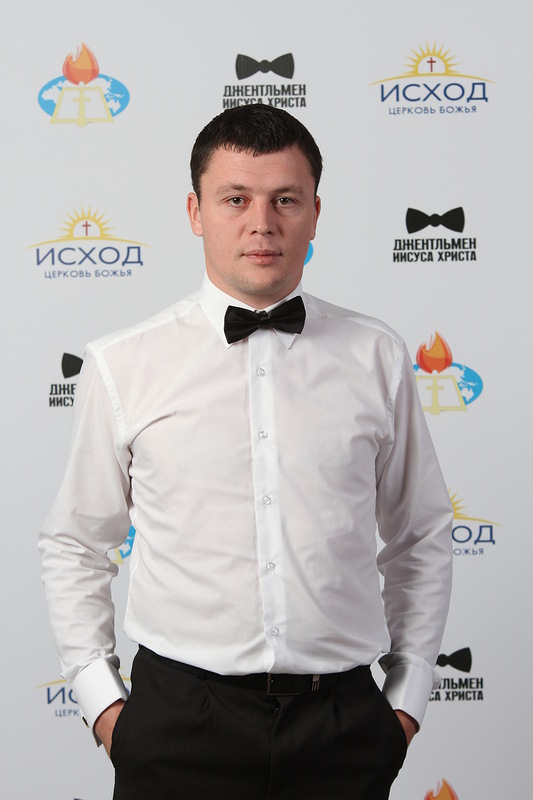In the center of the image, a well-dressed man stands, gazing directly into the camera with a serious expression. The man, with dark brown hair and brown eyes, wears a white button-down shirt, complemented by a black bow tie, black slacks, and a black belt with a silver buckle. His hands rest in his pockets, and the image cuts off a little below the waist.

Behind the man is a backdrop filled with various icons and ads, predominantly featuring black bow ties, church icons, and imagery suggestive of a starburst of yellow light emanating from a cross. Another prominent logo depicts a book with flames above it. The text accompanying these icons and ads is written in what appears to be Cyrillic script, repeated beneath each symbol.

The colors in the image range from black, white, and tan to accents of orange, yellow, and maroon. The setting is indoors, likely at a formal event, though the time of day is indeterminate. The overall composition centers on the man standing against this detailed and symbol-laden backdrop.